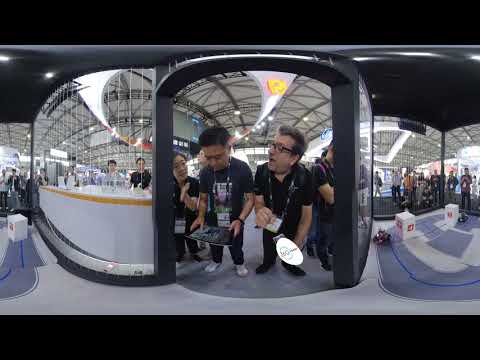This image portrays an indoor scene at an exhibition or convention, captured with a distorting lens that creates a panoramic and flattened effect. Central to the frame are four individuals who appear distorted but engaged with various electronic items. One man, dressed in a dark blue t-shirt, black pants, and white shoes, is holding a tablet. Another man, characterized by his short brown hair, black-framed glasses, black shirt, black pants, and black shoes, is standing nearby, seemingly focused on an item in his hand. Flanking them are two more individuals—the man on the left in dark clothing and white shoes, and another person, also in dark attire, whose oval-shaped item might be a result of the lens distortion. 

All individuals appear to be of Asian or Asian American descent, except for the man with brown hair. To the left and right of the central figures are glass booths with people in the middle and far distances, indicative of the event's large scale. The viewing angle from within a glass room emphasizes a larger structure, possibly a convention hall or airport area, bustling with attendees. The distorted perspective and dynamic positioning of the subjects give a sense of the event's vibrant atmosphere.